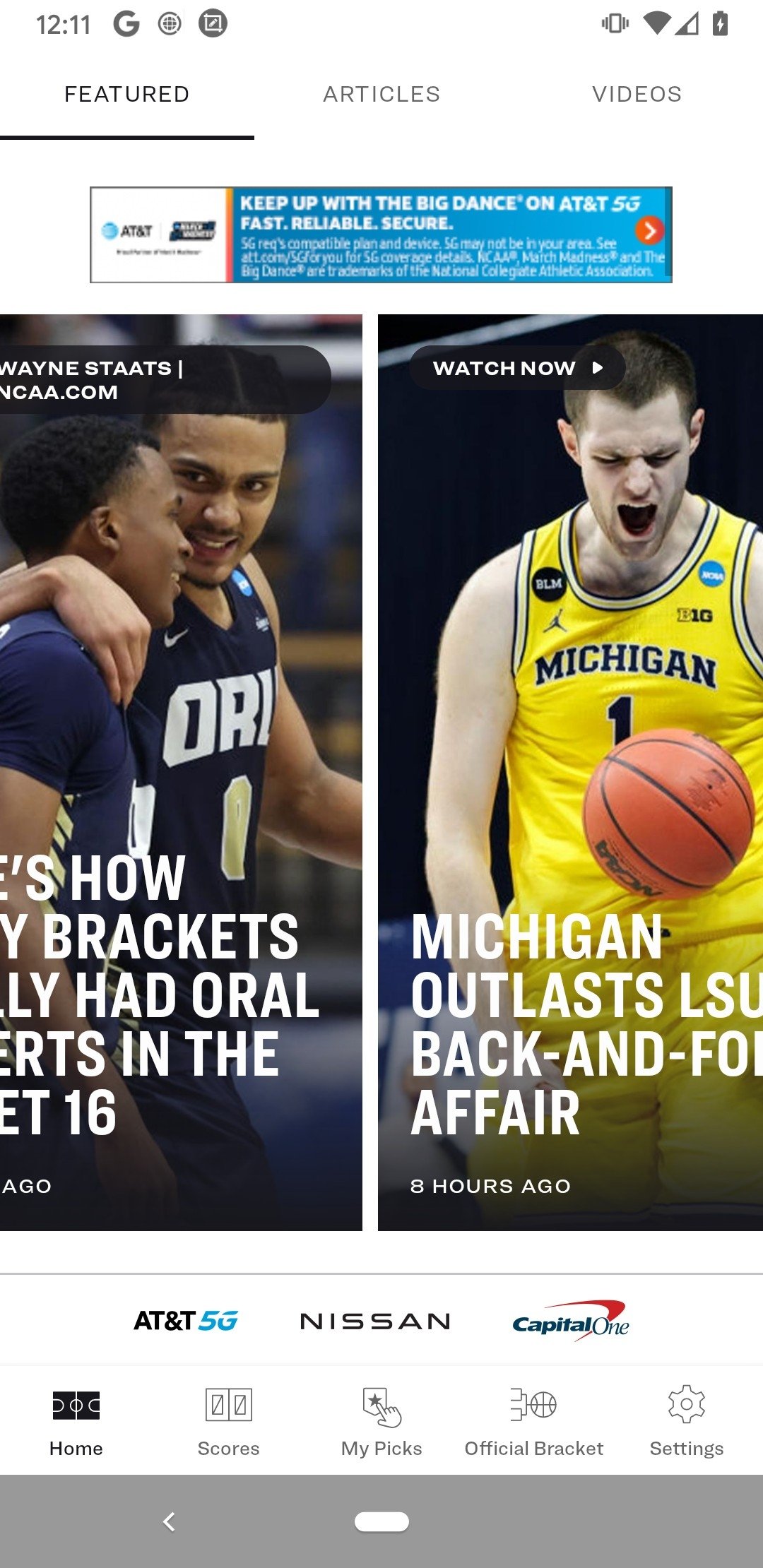Screenshot Description:

In this smartphone screenshot, the status bar at the top displays the time as 12:11. To the right of the time are several icons, including a Google "G" icon, an unidentified icon with boxes inside a square, another with boxes inside a circle, a crossed-out square within a circle, the cell carrier signal icon, the Wi-Fi icon indicating active connection, a battery icon showing approximately 50% charge, and finally, a camera icon.

Below the status bar, there is a navigation bar with three options: "Featured," "Articles," and "Videos." Underneath this bar is a clickable advertisement for AT&T. The main content section features two photographic images. 

The image on the left shows two basketball players, with one player's arm around the other. The text accompanying this image reads "WayneStats NCAA.com," with the rest obscured except for "how brackets had oral in the sweet 16." 

The image on the right features a basketball player from Michigan and captions reading "Michigan outlasts LSU back and forth affair," indicating the article was written eight hours ago. Both images appear to be clickable links.

Beneath these images are icons for advertisers including AT&T 5G, Nissan, and Capital One, displayed horizontally. Further down, there is another navigation bar featuring "Home," "Scores," "My Picks," "Official Bracket," and "Settings," all of which are clickable. At the bottom is a gray bar with a back arrow icon.